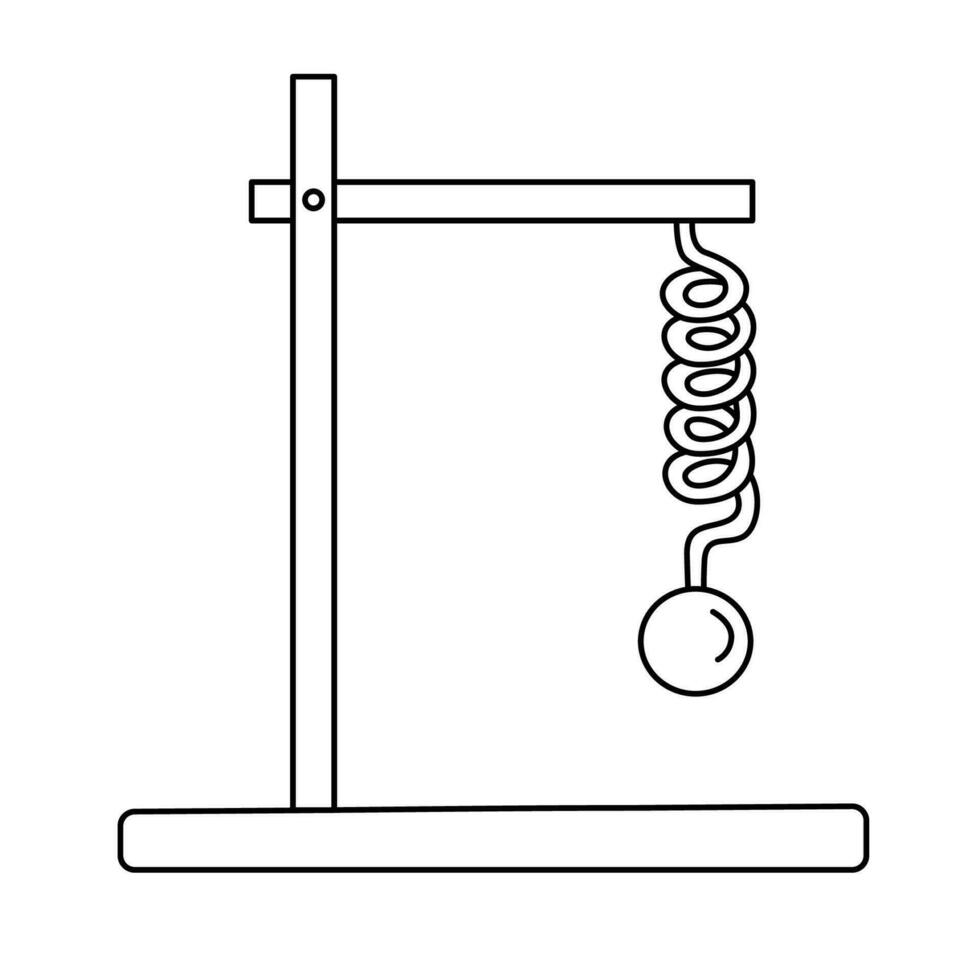This is a minimalistic, black-and-white illustration of an unidentified apparatus with a transparent background. The diagram features a long, rectangular base with smooth, rounded edges. Attached to the top of the base, there is a vertical post. Towards its upper section, closer to the center, another horizontal bar is secured to the post, likely fastened by a screw. Extending from the right end of the horizontal bar is a spiraling spring with five coils. The spring descends in a helical pattern, terminating in a small spherical object. The overall style is amateur and simple, with no photographic elements, text, people, animals, buildings, or motorized vehicles included in the image. The exact function of this spring apparatus is undetermined.